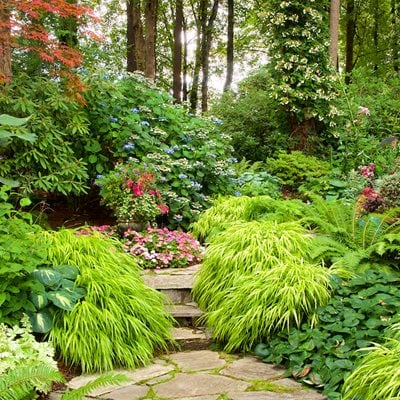The photo depicts a lush, verdant tropical garden brimming with vibrant foliage and colors. In the foreground, it features a flat, paved stone floor with tufts of grass peeking between the stones. Green vegetation and vibrant leaves surround this stone pad. Three stone steps ascend from the paved floor to a slightly elevated walkway. This pathway winds back to the right and is lined with a plethora of green leaves, bushes, shrubs, and ferns.

On the elevated level, there's a colorful flower bed that showcases pink, white, red, and blue flowers, adding a burst of color amid the greenery. Specific details include a white vine climbing a tree, and plants with large leaves featuring white centers. The rich assortment of plant life includes light green, dark green, and green with yellow-tinted leaves.

As the pathway progresses, it leads into a more densely vegetated area that resembles a forest. Tall tree trunks rise above this dense foliage, creating a canopy. In the distant background, the top center of the photograph reveals a bright, whitish-blue sky peeking through the dense greenery, giving the scene a sense of depth and tropical abundance.